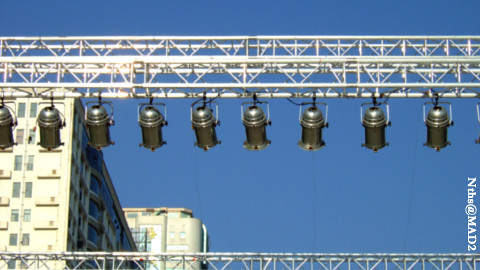This outdoor photograph captures a vivid scene under a royal blue sky. Dominating the background to the left, two tall buildings rise, with one prominently displaying a side view that features a vertical row of six large windows. The upper portion of the image showcases a horizontal lattice work or grid-like structure made of metal beams, from which dangle around nine lantern-like black spotlights. Each spotlight, equipped with a handle and metal top, points down, suggesting they are designed to illuminate a nighttime event. Below, a similar metal structure spans horizontally from left to right. In the right-hand corner, the text "NTHS at MAD2" overlays the image in white lettering, adding a distinct element to the composition.